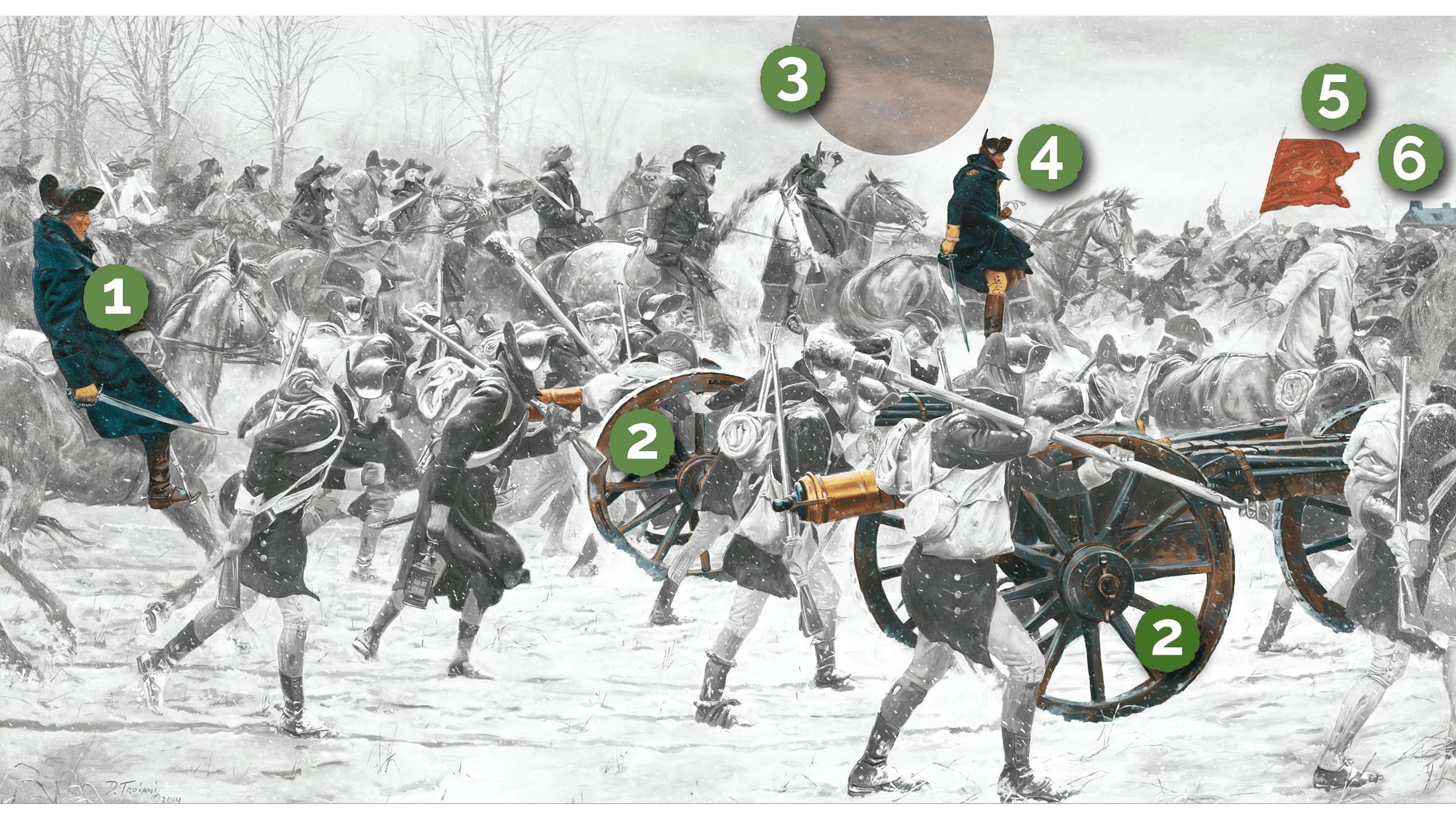This image depicts a detailed and historically themed scene of a Napoleonic-era battlefield. It features soldiers and artillery amidst a march, with notable elements highlighted by numbering. The image predominantly presents in grayscale, with six distinct colorized portions:

1. A general in a blue coat mounted on a horse.
2. A cannon wheel.
3. Part of the sky.
4. Another rider on horseback wearing a French-style hat typical of the Napoleonic era, carrying a musket.
5. A red flag.
6. An indistinct blue-colored structure in the distance.

The scene showcases a mix of mounted cavalry wielding swords and carrying muskets, as well as artillery units with primitive breech-loading cannons. The artistry captures the essence of an early 19th-century military spectacle with attention to period-specific details.